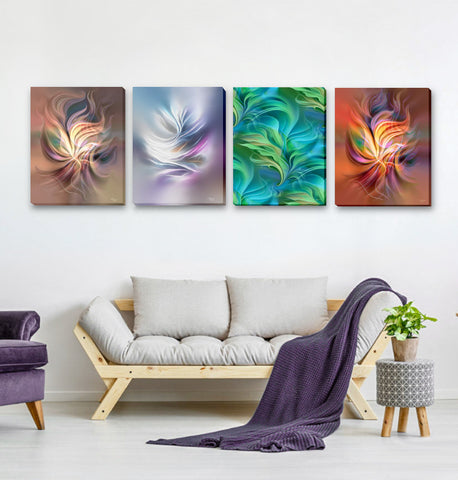In this modern interior design-themed image, a cozy living room or office area is depicted with a serene, monochromatic backdrop, where both the wall and floor blend seamlessly in a light beige/white tone. Central to the composition is a two-seat loveseat boasting a wooden base and comfortable, off-white cushions—including quilted ones on the bottom and sides. Draped diagonally over the right side of the loveseat is a dark purple throw blanket, adding a touch of color and warmth.

To the right of the loveseat, there’s a planter stand featuring intricate patterns, balanced on three wooden legs, with a lush plant in a brown container perched above it. On the left side, a sleek, grey coffee table hosts a plant, complementing the loveseat’s modern aesthetic.

Dominating the wall above the loveseat are four square canvases, each showcasing abstract, wavy floral patterns with blurred edges. The artwork ranges in color, transitioning from a warm pink, purple, and yellow palette on the far left, to a cooler white, purple, and blue design. Next in line is a predominantly green and turquoise piece, culminating in a vibrant reddish-orange and purple canvas on the far right. All these elements together create a harmonious and inviting space, marrying modern furniture with artful decorations.